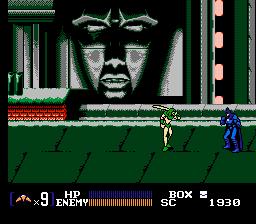In this image, we see a detailed screenshot from a video game displayed on a computer screen. The game appears to be a fighting game featuring a vibrant, grassy battleground. Two cartoonish characters are engaged in combat, with one character dressed in blue and the other in white and green. In the background, there is a wall adorned with a green and white mural, which includes a painted face. Additionally, health bars for both characters are visible at the top of the screen, each one fully filled, indicating that neither character has taken significant damage yet. The overall scene captures a moment of intense action set in a vividly illustrated environment.